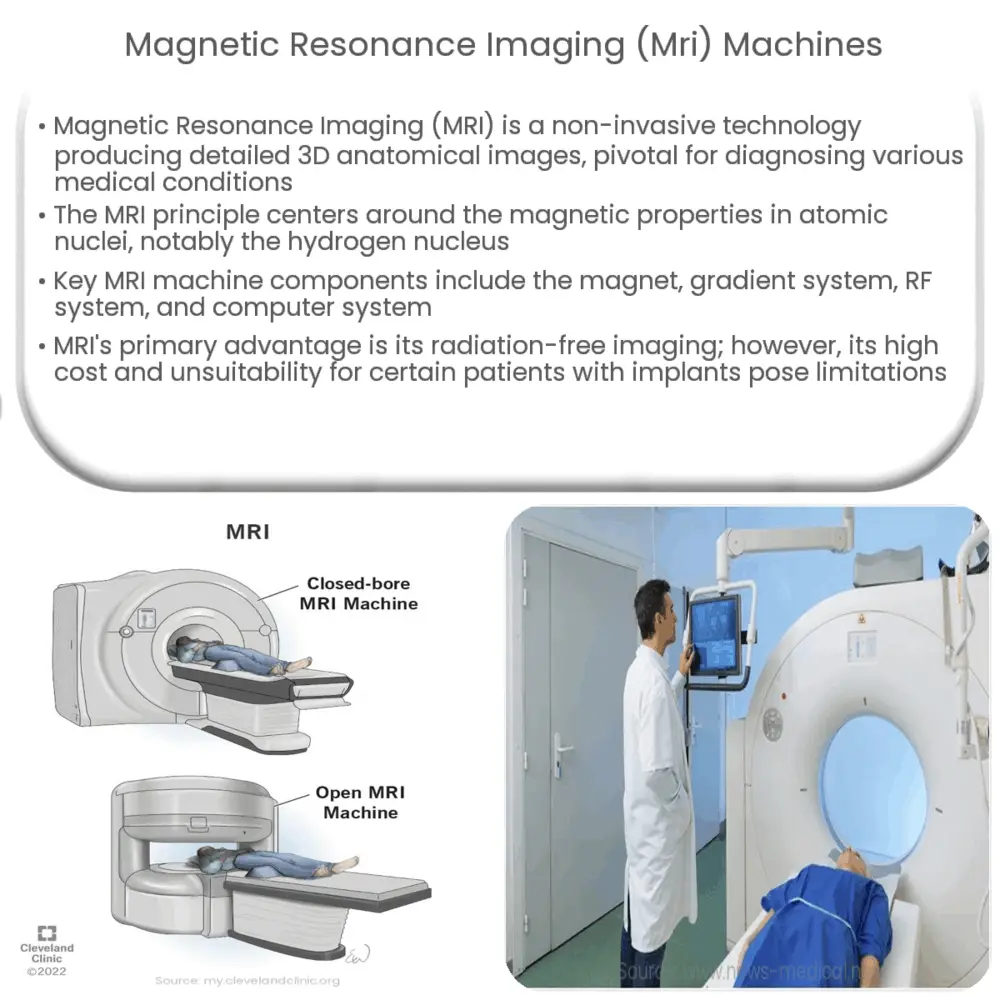The image is a detailed representation of Magnetic Resonance Imaging (MRI) Machines, with comprehensive textual and visual information. At the top of the image, "Magnetic Resonance Imaging (MRI) Machines" is prominently displayed in black letters against a white background. Below this title are four informative paragraphs describing the MRI, including its non-invasive technology that provides detailed 3D anatomical images crucial for diagnosing various medical conditions. The descriptions delve into the MRI's principle centered around the magnetic properties in atomic nuclei, especially hydrogen, and outline the key components such as the magnet gradient system, RF system, and computer system. It also highlights the primary advantage of MRI—radiation-free imaging—while noting the limitations due to high cost and incompatibility with certain implants.

On the left lower quadrant, there are two diagrams depicting different types of MRI machines. The upper diagram shows a body lying on a table labeled "Closed-Bore MRI Machine," illustrating a more enclosed structure. Below it, a diagram labeled "Open-Bore MRI Machine" shows a more spacious variant, emphasizing increased openness. To the right, in a color photograph, a patient in a blue hospital gown lies on a flat table, poised to enter a white MRI machine. A clinician, dressed in a long white lab coat, stands nearby examining films on a screen hanging from a metal fixture attached to the ceiling.

This detailed combination of text and images provides a thorough understanding of MRI machines and their operational context.